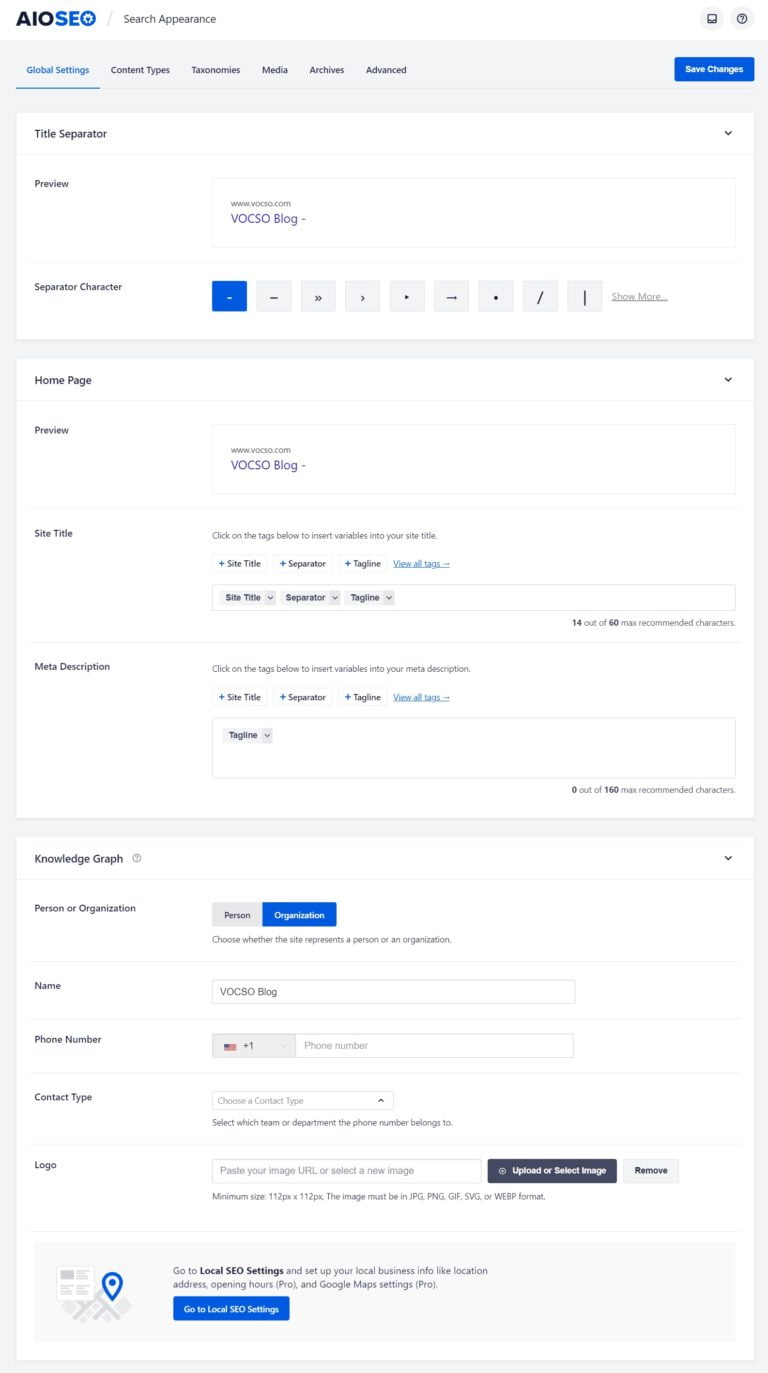**Screenshot Description: AIOSEO Global Settings Interface**

The screenshot displays the user interface of the AIOSEO (All-In-One SEO) plugin for a website, specifically in the "Global Settings" menu. 

**Top Left Corner:**
- The company name "AIOSEO" is prominently displayed, with "AIO" in black capital letters and "SEO" in blue capital letters.

**Menu Navigation:**
- Below the company name, the navigation path reads "Search Appearance."
- The selected menu item is "Global Settings," with other menu options listed as "Content Types," "Taxonomies," "Media," "Archives," and "Advanced."

**Main Section:**
- A blue rectangle labeled "Save Changes" in white letters is present, likely to save any modifications made on the page.

**Title Separator Section:**
- It features a "Title Separator" selection tool, with a preview URL "www.VOCSO.com — VOCSO blog."
- Different separator characters are shown, including:
  - A short dash (selected),
  - A long dash,
  - Two arrows pointing to the right,
  - One arrow pointing to the right,
  - A full arrow pointing to the right,
  - A dot,
  - A slash '/' and
  - A vertical line '|'.
- An option to "Show More" for additional separators is also available.

**Homepage Section:**
- Displays another preview URL: "www.VOCSO.com — VOCSO blog."
- Instructions to click on tags below to insert variables into your site title and meta description:
  - For "Site Title":
    - Tags: "Site Title," "Separator," and "Tagline."
    - Character count: 14 out of 60 max recommended characters.
  - For "Meta Description":
    - Similar tag options.
    - Character count: 0 out of 160 max recommended characters.

**Knowledge Graph Section:**
- A toggle to choose whether the site represents a "Person" or an "Organization" with "Organization" selected.
- Additional fields for:
  - Name: "VOCSO blog",
  - Phone Number: Includes an American flag icon and a prefix "+1",
  - Contact Type: Dropdown to select the relevant team or department affiliated with the phone number.
  - Logo: Option to paste the image URL or upload/select a new image. Provides constraints like minimum size (112px by 112px) and acceptable formats (JPEG, PNG, GIF, SVG, or WEBP).

**Local SEO Section:**
- Prompts to "Go to local SEO settings" to set up local business information, including location, address, opening hours, and Google Maps settings, with some features marked as "pro."

This detailed caption covers all visual elements and functionality present in the screenshot of the AIOSEO plugin's Global Settings interface.